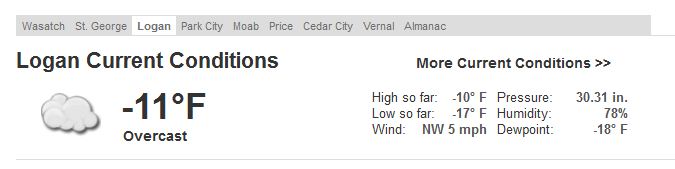**Caption:**

A comprehensive screenshot from a weather service website displays various selectable areas in tab format at the top. The tabs include "Wasatch," "St. George," and "Logan," with "Logan" being presently selected. Other tabs list "Park City," "Moab," "Price," "Cedar City," "Vernal," and "Almanac." 

Under the "Logan" tab, current weather conditions are detailed, featuring a cloud icon indicating overcast skies. The temperature reads -11°F. On the right side of the image, further current conditions are provided: the high temperature so far is -10°F, the low is -17°F. Additionally, the wind is coming from the northwest at 5 miles per hour, atmospheric pressure is noted at 30.31 inches, and humidity is at 72.18%.